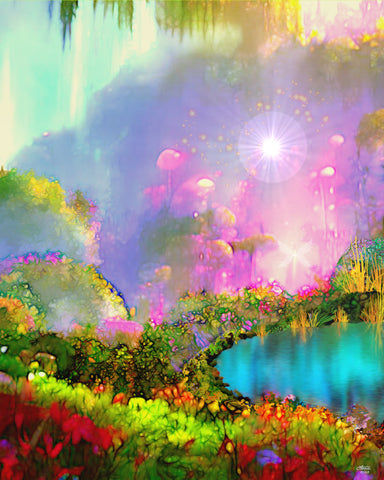The image is a vibrant, whimsical painting of an enchanting glade that evokes a fairy-tale atmosphere with its psychedelic colors and mystical details. The foreground is dominated by lush green leaves and grass, interspersed with brightly colored flowers ranging from pink and orange to purple and blue. On the right side of the painting lies a shimmering, turquoise lake that reflects its surroundings.

In the lower left corner, red flowers bloom among green bushes, leading the eye towards opalescent water. Above this enchanted scene, the trees are adorned with hues of purple, pink, and yellow, and their canopy is punctuated by leaves resembling those of a weeping willow, painted in vivid greens.

The background features an ethereal glow with shades of orange and pink, originating from what appears to be a radiant orb or sun located towards the middle right. This orb emits white light with a halo, casting rays that illuminate the sky, which transitions into blue with white streaks across the upper left.

Moreover, a dragonfly flits about amid various flora, including mushrooms and mopey willow trees, adding to the enchanting, otherworldly allure. The overall composition is rich in detail, inviting viewers to lose themselves in its multitude of hidden elements and phantasmagoric beauty.